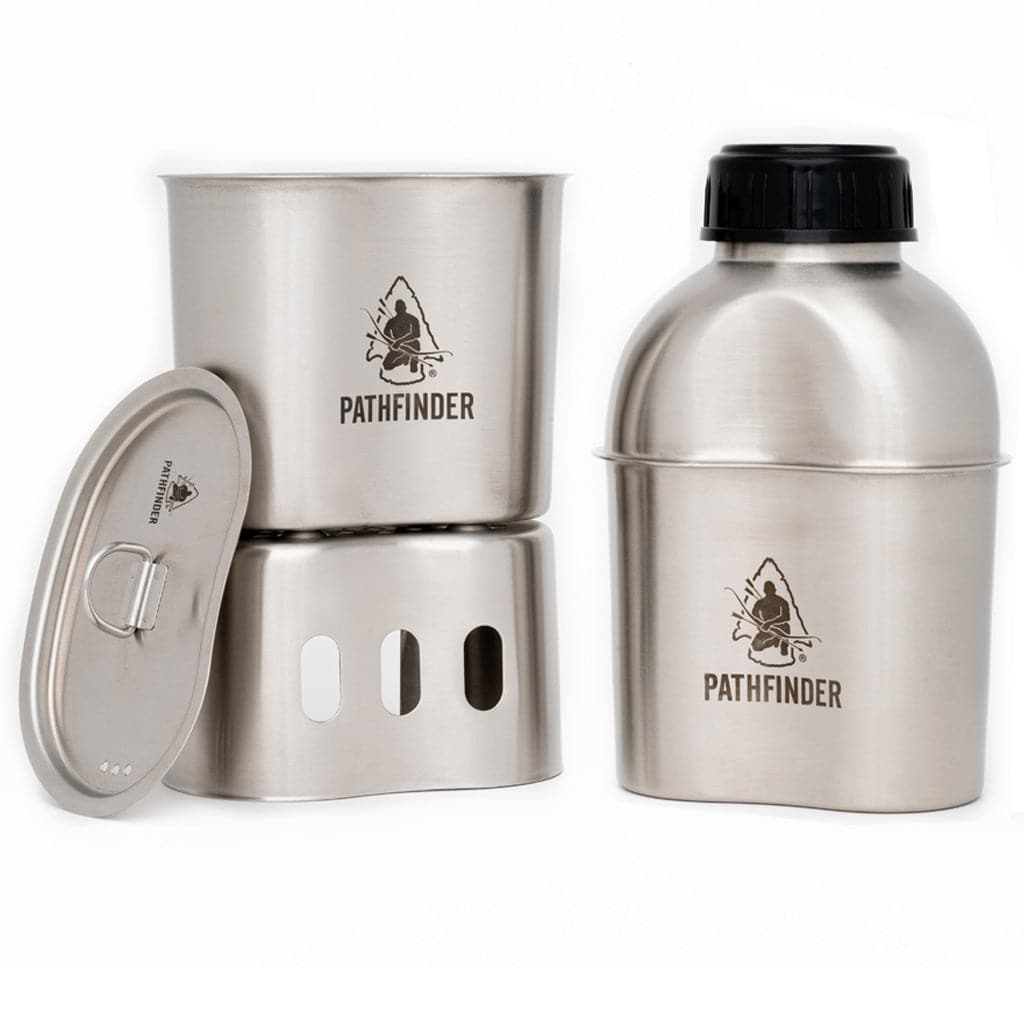This image showcases a stainless steel canteen product designed for camping, prominently featuring the Pathfinder logo. The logo depicts a man squatting, overlaid on the silhouette of an arrowhead. The canteen is comprised of two main sections: the primary body and a curved upper part, topped with a black plastic cap. The image displays the canteen twice side by side; the canteen on the right is assembled with the cap on, while the canteen on the left is disassembled, revealing the bottom part set on a stainless steel piece which resembles a portable cooking unit. This unit appears to have small holes for ventilation, suggesting it may be used to heat food or boil water, ideal for outdoor activities like camping. The setup includes a lid placed next to the bottom section, further highlighting its functionality as both a water carrier and a compact portable stove.